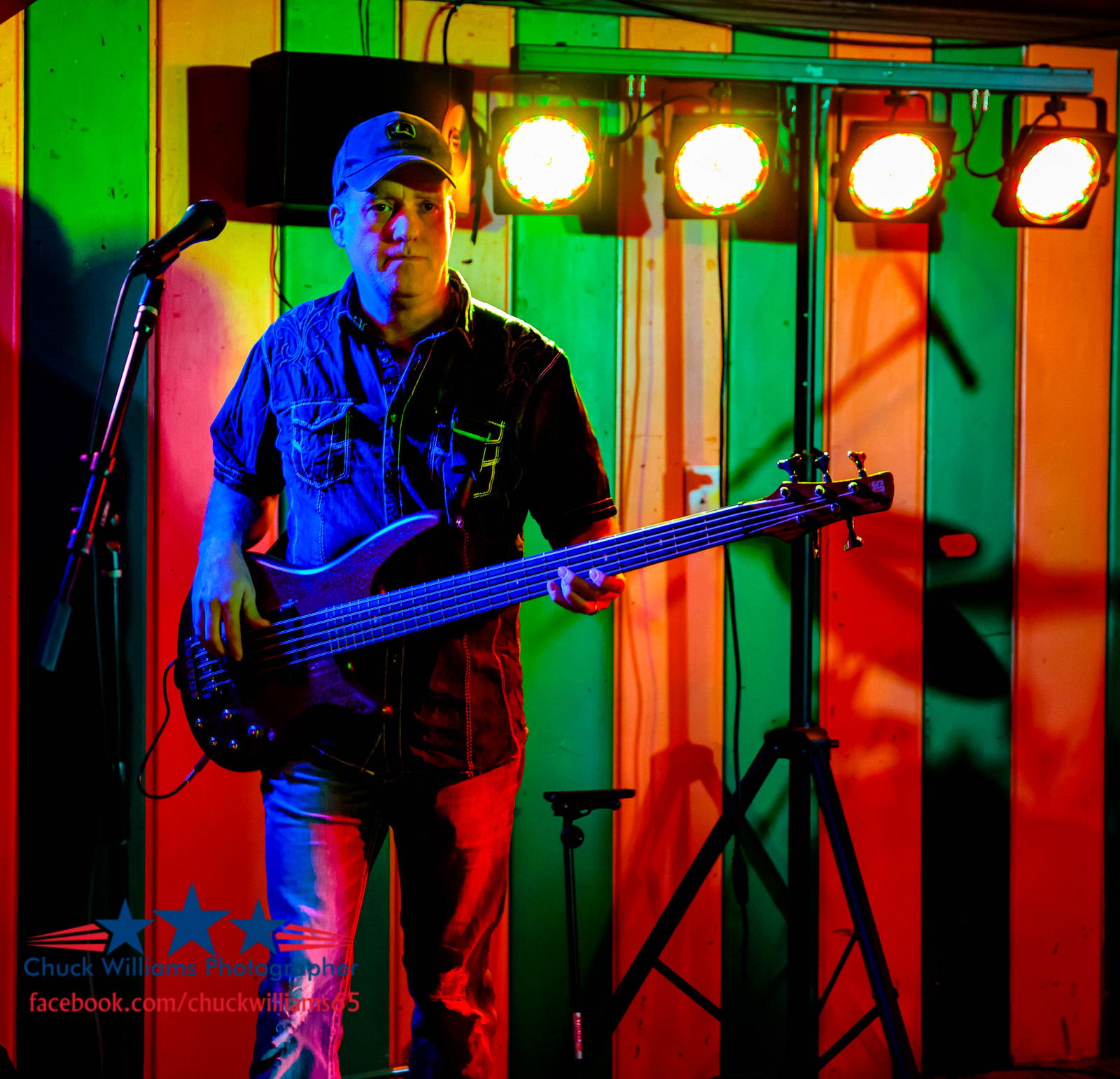In this vivid and close-up image, a man, likely around 45 years old, stands at the foreground holding a blue guitar. He is dressed in a blue short-sleeved shirt, blue cap, and jeans, and appears to be staring intently ahead. Behind him, the wall is adorned with alternating green, yellow, and orange striped patterns, giving a lively backdrop. To his left, there's a black standing microphone and to his right, a three-legged stand supporting four circular white spotlights. Situated at the lower left of the image, a logo with three horizontal pink stripes, three blue stars, and again three horizontal pink stripes prominently features the text "Chuck Williams Photography." Below this logo, the text "facebook.com/ChuckWilliams65" can be seen. The overall scene suggests a promotional photograph, possibly captured in a stage-like setting.